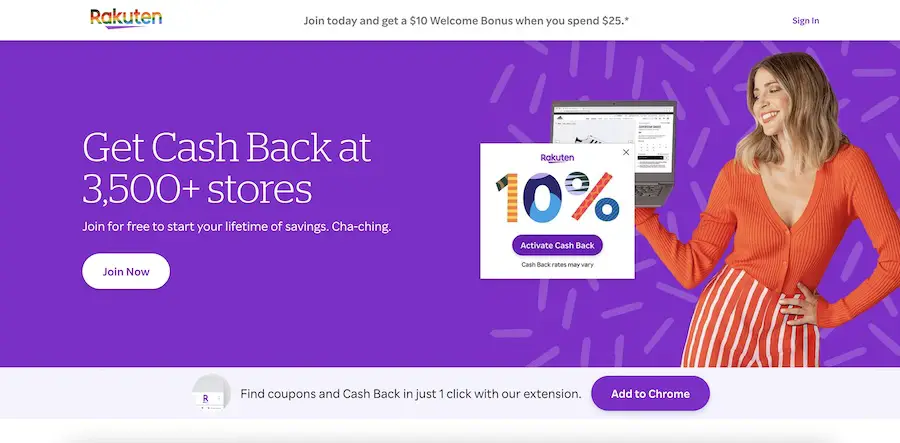Screenshot of a Rakuten Desktop Advertisement

In this Rakuten advertisement screenshot, observed from a desktop interface, the Rakuten logo is prominently displayed at the top left corner, adorned with its vibrant Pride Month variant. At the center-top section of the screen, a banner exclaims, "Join today and get a $10 welcome bonus when you spend $25," accompanied by a convenient sign-in button situated on the right.

The main visual content boasts a purple background. To the right, a smiling woman, clad in bright orange attire, holds a laptop. Overlaying this image is a prominent message proclaiming, "Rakuten 10% activate cashback, cashback rates may vary."

On the left side, a bold headline reads, "Get cashback at 3,500+ stores," followed by "Join for free to start your lifetime of savings, cha-ching!" Beneath this engaging text, a conspicuous "Join Now" button invites immediate interaction.

At the very bottom of the screen, an enticing prompt states, "Find coupons and cashback in just one click with our extension," complemented by a purple "Add to Chrome" button, seamlessly integrating enhanced convenience with compelling incentives.